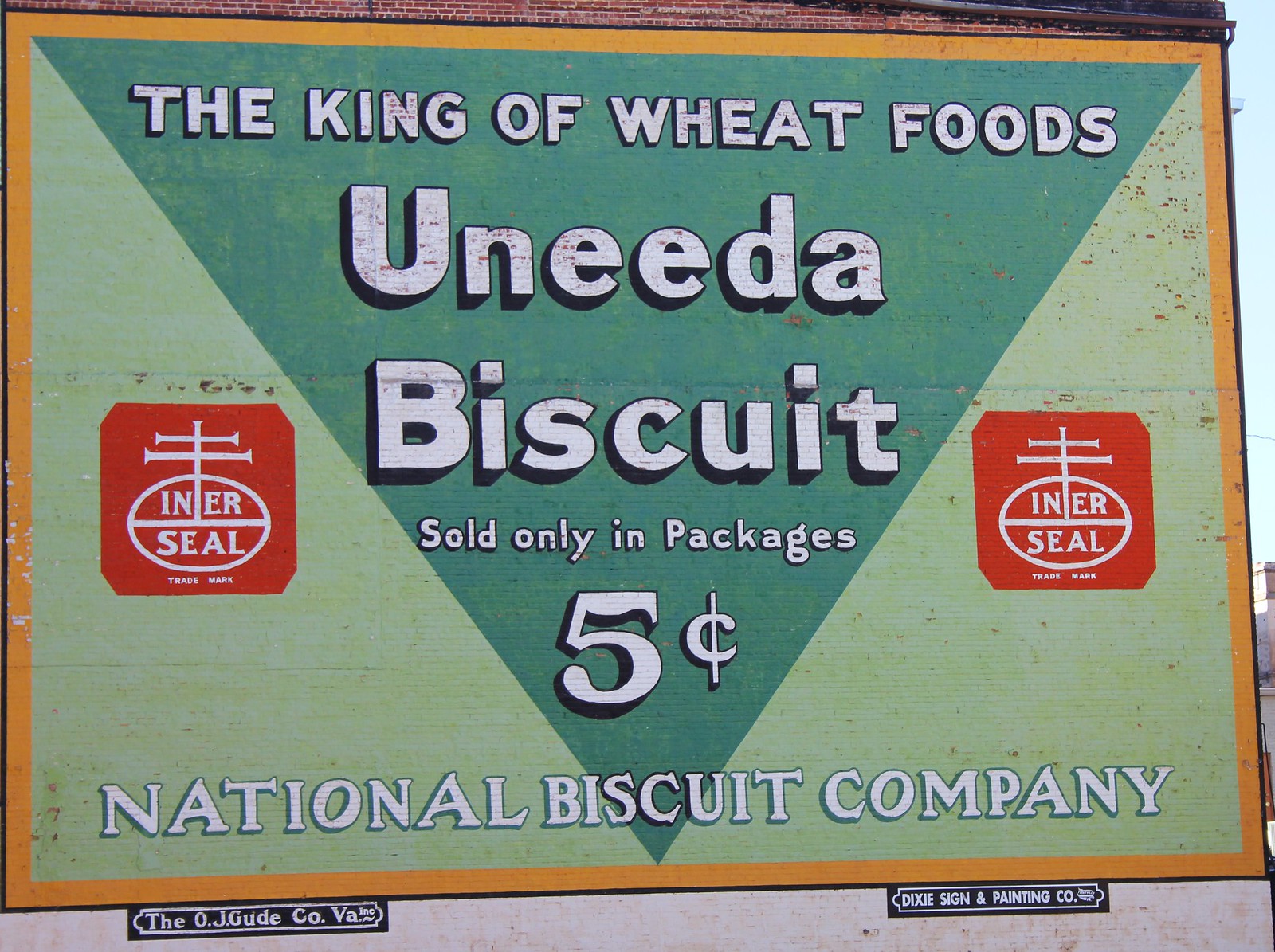This photo captures a detailed mural painted on the side of a brick building. The image is bordered by a yellow frame that encloses a dual-toned background with a light mint green hue and a darkish green inverted triangle at the center. The mural prominently features bold white letters edged in black, reading: "The King of Wheat Foods, You Need a Biscuit." Directly beneath this, it declares: "Sold Only in Packages, Five Cents." 

Both the left and right sides of the dark green triangle host red squares containing identical circular icons with white text stating "Inner Seal." A distinctive cross-like shape appears behind the text within these circles. The name "National Biscuit Company" is prominently displayed in white letters at the bottom of the mural.

Additional text at the bottom credits "The OJ Good Co. VA" and the "Dixie Sign and Painting Co." The sign, facing a shaded part of the building, depicts a classic advertisement style reminiscent of the Nabisco seal, exuding vintage charm and possibly a touch of humor.